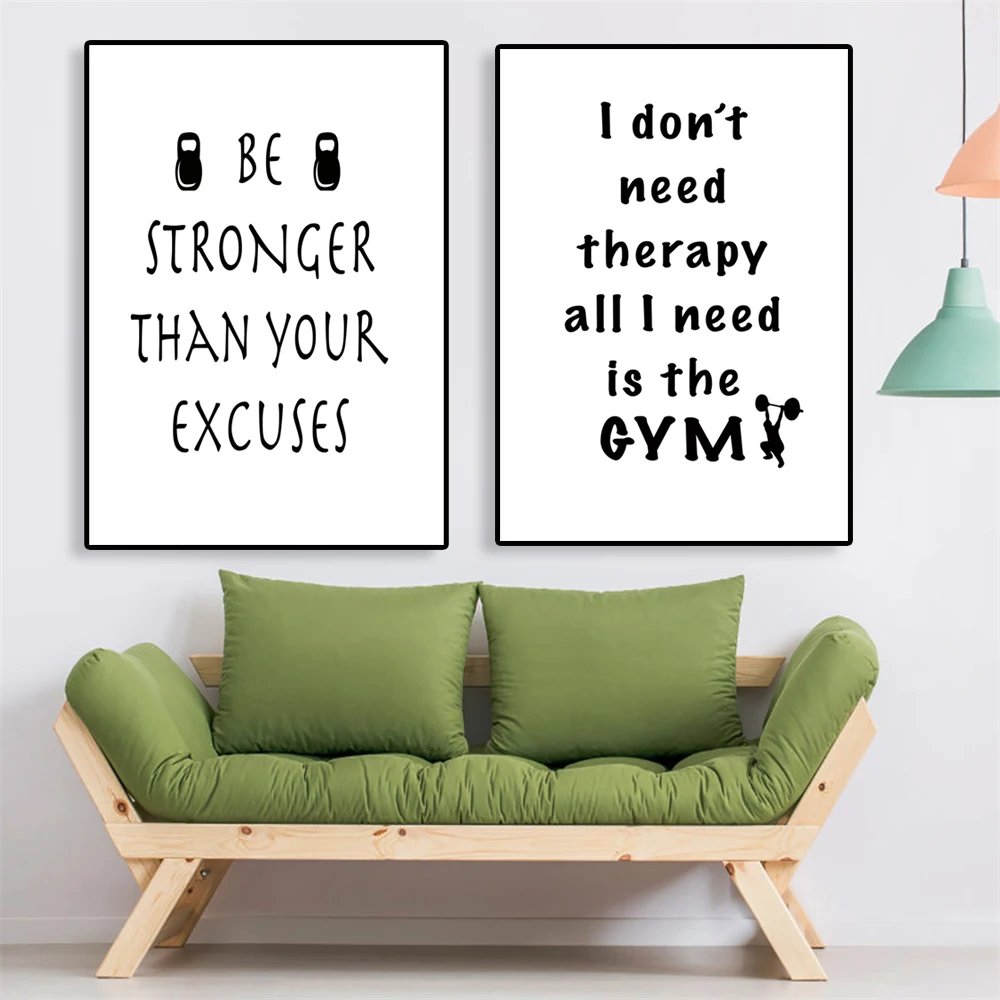The image showcases a meticulously arranged, bright living room that evokes a modern, minimalist aesthetic. At the forefront is a sleek, oak-framed sofa adorned with green cloth-like cushions and two matching rectangular pillows. The sofa is designed akin to a futon, with its wooden structure providing a balanced contrast to the soft, earthy green cushions. 

Above the sofa, the white gradient wall serves as a backdrop for two framed motivational posters. The left poster, slightly larger than its counterpart, boldly declares "BE STRONGER THAN YOUR EXCUSES" in a prominent, all-capital font, flanked by kettlebell icons. The right poster, differentiated by its use of varied fonts, reads "I DON'T NEED THERAPY. ALL I NEED IS THE GYM," with "GYM" emphatically bold and uppercase, accompanied by a vector graphic of a man squatting with a barbell.

To the right of these posters hang two pendant desk lamps, one in a soft seafoam green and the other in a warm peach hue, adding subtle pops of color. The floor beneath the scene is a modern, grayish linoleum finish that complements the clean, white walls and overall contemporary design of the room. This carefully styled setup suggests an advertisement for furniture or home decor, focusing on the couch and inspirational wall art.